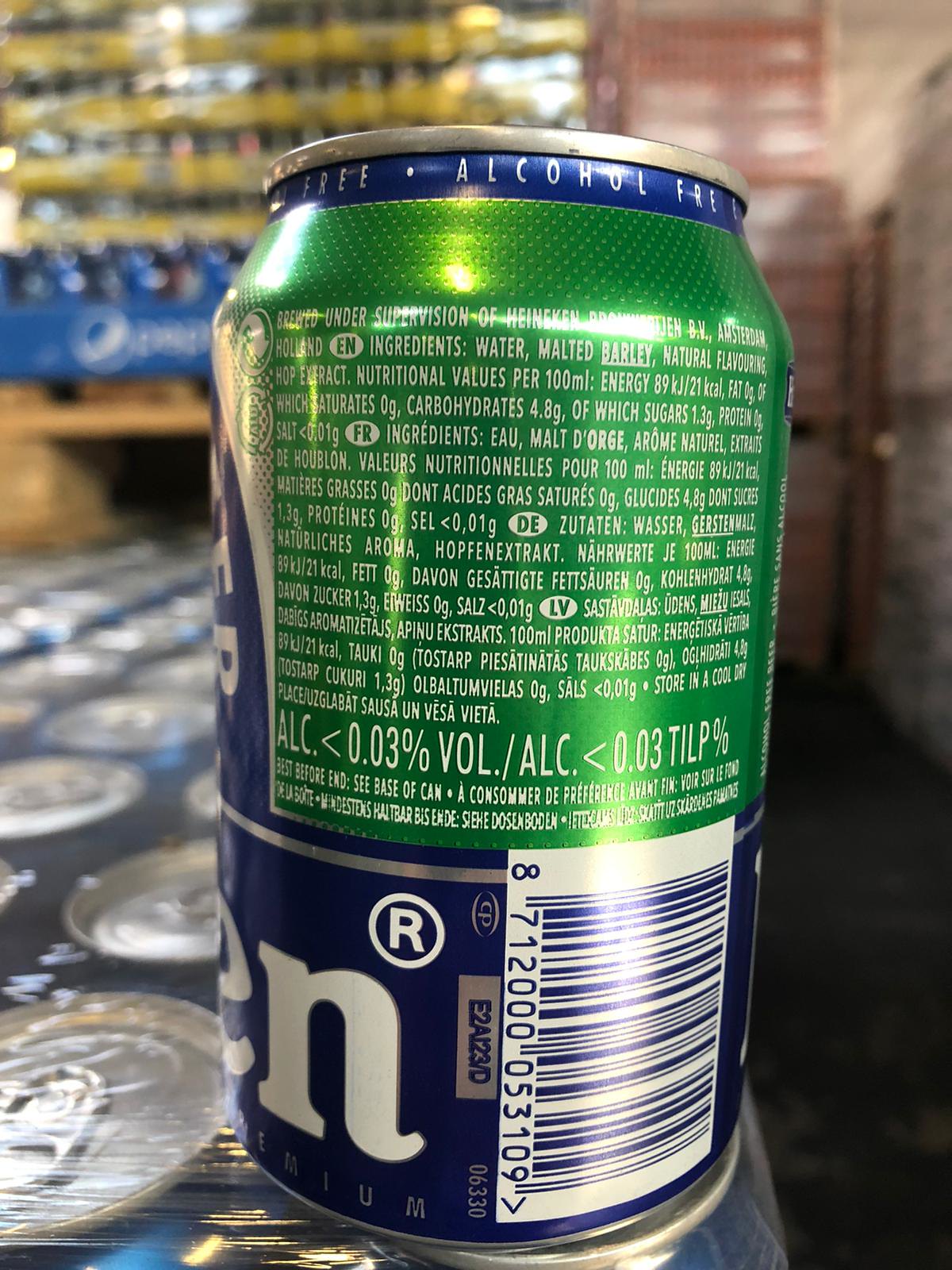The image features a close-up of the back of a Heineken non-alcoholic beer can, distinguished by its iconic bright green and blue color scheme. Prominently displayed at the top, just below the lip of the can, are the words "alcohol-free." The detailed backdrop reveals a warehouse or stockroom setting, with boxes and pallets of drinks, including Pepsi bottles, stacked high. The can appears to be placed atop blue plastic-wrapped drink pallets. The Heineken can displays its nutritional facts and ingredients, such as water, malted barley, and natural flavoring, in multiple languages including English, French, and Dutch. Notably, the label indicates an alcohol content of less than 0.03 percent. A barcode is visible at the lower right of the can.